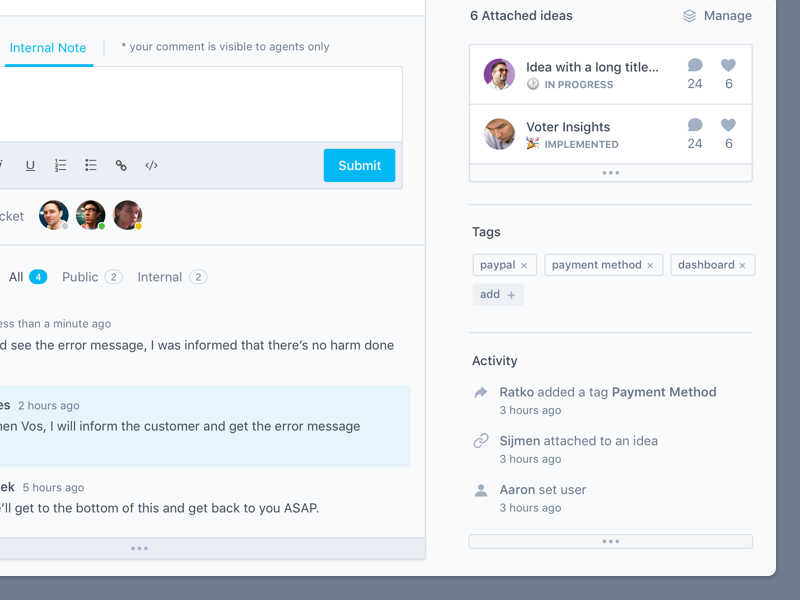The image depicts a digital interface seemingly from a customer support or internal communication platform. The top left corner features a label "Internal Notice." Adjacent to this label, there is a message area where users appear to be exchanging internal comments. Accompanying text indicates that any comments made here are visible only to agents, signified by the phrase, "Your comment is visible to agents only.” Below this main text area, a blue submit button is set against a gray background strip.

Further below, there are bullet points formatted in both numerical and circular styles, seemingly to outline various points or steps. The interface also shows three round profile pictures, each slightly indicating different statuses labeled as "Public" or "Internal," followed by respective indications of time, such as "less than a minute ago." 

However, the actual conversation cut-off occurs on the left side, rendering it difficult to read the entire context. Visible portions of the conversation include statements like:
- "See the error message I was informed that there were no there's no harm done."
- Other segments include, "This is two hours ago. I will inform the customer to get the error message."
- Earlier messages include, "Five hours ago. I'll get to the bottom of this and get back to you ASAP."

On the right side of the interface, six attached ideas are listed in a straightforward manner:
1. "Manage idea with long title (In Progress)"
2. "Voter Insight (Implemented)"

Each idea entry appears to be interactive, possibly allowing for additional actions or comments. Below these entries are their individual statistics, such as "24 comments" and "6 likes."

Near the bottom, a tagging system is visible, indicating various categorized elements like "PayPal," "payment method," "dashboard," "add activity," and "rato," which seem relevant to the context of conversations or ideas being managed.